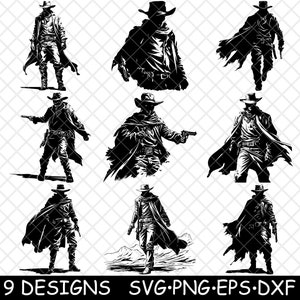In the image, there are nine different black and white illustrations of a cowboy laid out on a grey and white checkerboard background. All the cowboys are dressed in hats and varying attire, including capes or ponchos, with some images showing them holding guns. On the top left, the cowboy is simply standing, while in the middle top image, there's a half-body shot. The top right shows the cowboy walking, holding a gun in his left hand. The middle row features the cowboy aiming his gun on the left, pointing his weapon directly ahead in the center, and having his hands in his pockets on the right. In the bottom row, the left image depicts the cowboy standing with a gun at his side, the middle image shows him walking, and the right image has him holding the weapon at his side again. The cowboy's facial features are obscured by either a bandana or shadow from his hat in all images. The designs are annotated with a black bar at the bottom, stating "nine designs SVG, PNG, EPS, and DXF."